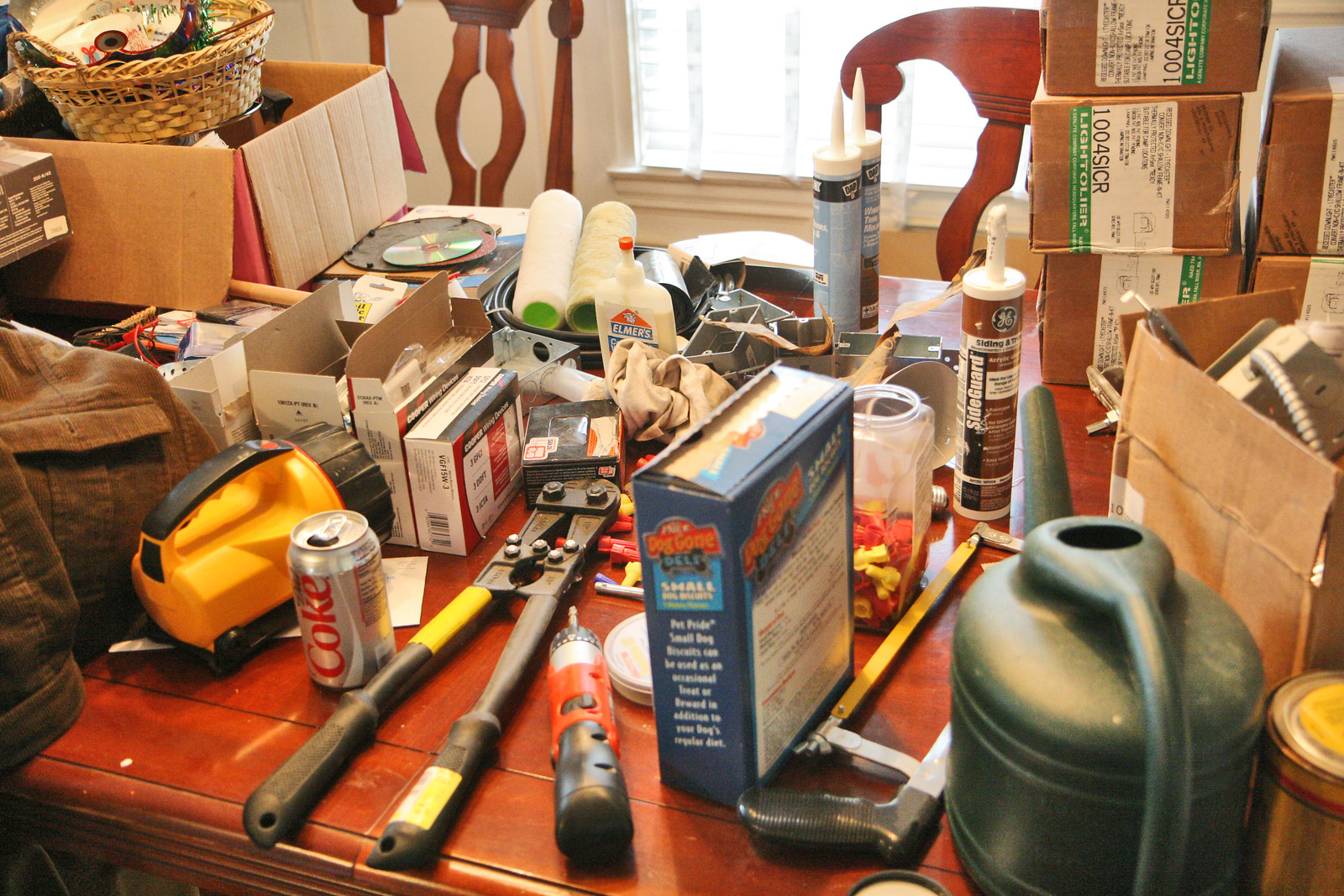The photograph showcases a well-worn wooden table surrounded by an array of tools and supplies. On the table, several cardboard boxes can be seen; some are closed and neatly stacked atop one another, while others are open, revealing their contents. Among the items stored in and around the boxes are three upright tubes of sealant, a large set of pliers, a hefty wrench, and a metal handle. A cordless screwdriver and a saw lie nearby, alongside long spools of string and a white plastic tube of Elmer's glue. Additionally, baskets filled with fabric are spread across the table. Prominently displayed is a big yellow torch with a black handle, and a folded brown jacket rests casually to the side, completing the scene of organized clutter.